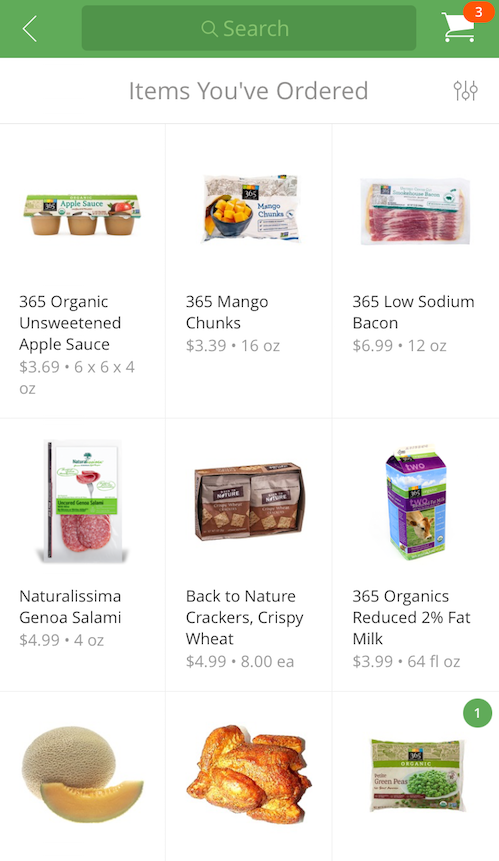The website features a dark green header at the top. Below this header, the background is white. In the top left corner, there is a white "greater than" symbol pointing left. Approximately half an inch to the right of this symbol, there is a darker green search bar that spans nearly the entire width of the page. Inside the search bar, there is a white search icon accompanied by the word "Search."

In the top right corner of the header, a white shopping cart icon with its handle facing left is displayed. A red circle containing the number "3" is located at the top right corner of the shopping cart icon. 

Below the header, in the center of the page, blackish text reads "Items You've Ordered." Below this heading, three vertical lines are displayed: the first line has a small circle at the top, the second line a circle at the bottom, and the third line a circle at the top again. There is a horizontal line halfway down the vertical space, and another horizontal line an inch from the bottom. This section is divided into thirds by thin gray lines, both vertically and horizontally, creating a 3x3 grid with nine sections in total.

Each section contains an image at the top, followed by the product name in black text, the price in a lighter gray-black text, and the quantity and unit below that. For example, the first section on the top left displays an image of 365 Organic Unsweetened Applesauce. Below the image, the text reads "365 Organic Unsweetened Applesauce," followed by the price "$3.69" and the quantity "6 x 4 ounce."

The bottom row sections display only images of items, except for the last one on the bottom right, which also has a green circle with a white number "1" inside it.